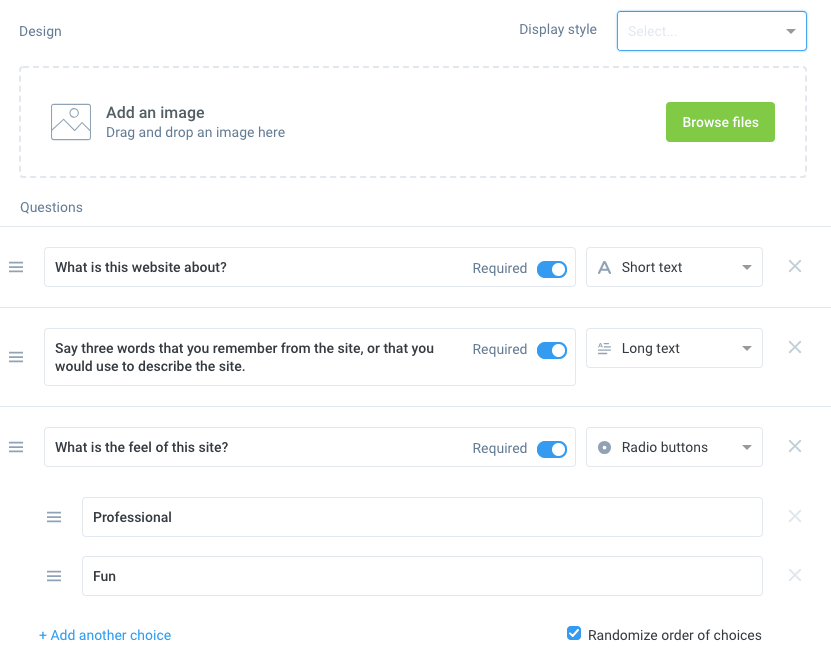The image depicts a user interface, likely from a website or an application, dedicated to building quizzes or tests. The overall aspect ratio is slightly wider than it is tall, although this is estimated due to the lack of clear borders. 

In the top left corner, the word "Design" is displayed in small, gray text. Adjacent to it, the term "Display Style" is presented, followed by a blue dropdown box containing a faint "Select" and accompanied by a gray downward arrow.

Directly below this section, there's a rectangular area outlined with a dotted gray line. Inside this area, instructions read, "Add an image, drag and drop an image here," aligning to the left. On the right side of this rectangle, a green button labeled "Browse Files" invites users to upload an image.

Further down, another header titled "Questions" appears on the left side, identical in alignment to the previous "Design" header. A horizontal line stretches beneath this header from left to right. Below this line, a menu icon consisting of three horizontal lines is positioned on the left. To its right, a box contains the question, "What is this website about?" in black text. To the right of this text box, a toggle switch labeled "Required" is set to the 'on' position.

Given these elements, the layout suggests that the interface is part of a quiz or test creation tool, guiding users through the process of designing questions and incorporating images.